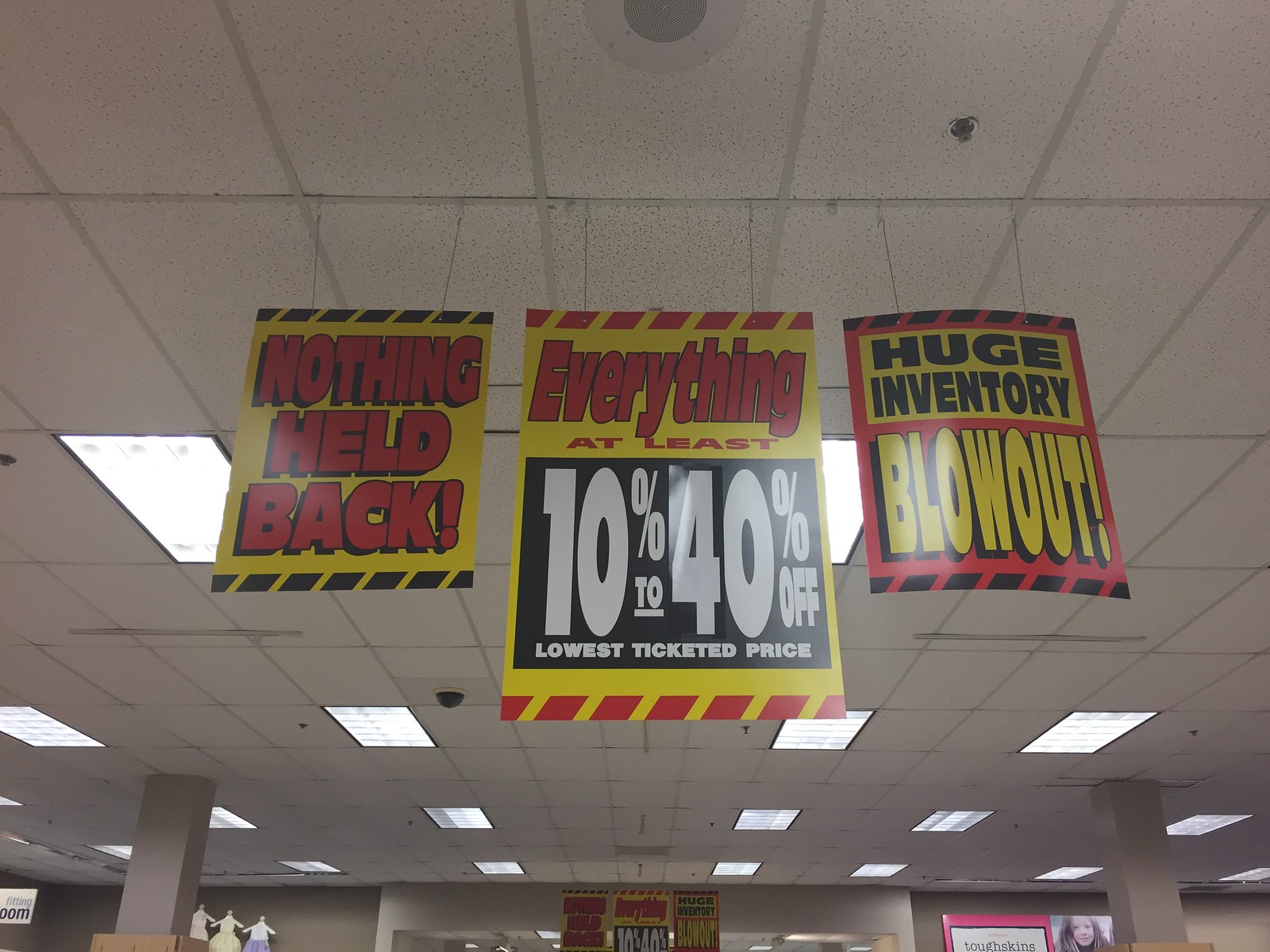The image depicts the interior of a retail store with a drop ceiling featuring long rectangular white tiles and fluorescent lights. Several smoke alarms and a security camera are visible on the ceiling. The store appears to be in the process of closing, as indicated by prominent signage hanging from above.

On the right-hand side, a yellow sign with black and yellow stripes along the top and bottom edges reads, "Nothing Held Back" in large red letters. The central sign is the longest of the three and features a red and yellow stripe at the top. It states "Everything" in large red letters, followed by "at least" in smaller red letters and "10% to 40% off lowest ticketed price" in white letters on a black background. This sign seems designed for flexible messaging, allowing for further updates to the discount levels. 

The third sign, on the left-hand side, is the same size as the first. It is red and reads "Huge Inventory Blowout" with "Huge Inventory" in black letters enclosed in a yellow rectangle, and "Blowout" in yellow letters.

The background indicates that the store likely sells clothing, as evidenced by three child-size mannequins situated in the back right corner next to a pillar. Additional signs and another pillar can also be seen further back in the image.